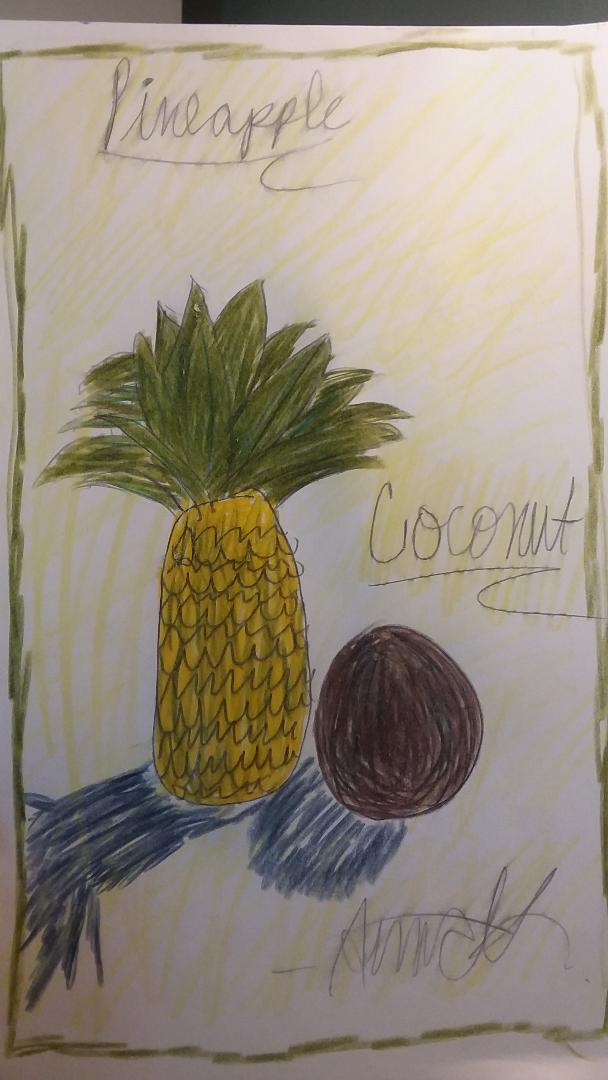The image depicts a vibrant homemade drawing on a rectangular, vertically oriented piece of paper. At the center of the artwork is a yellow pineapple with green leaves sprouting from its top. The texture of the pineapple is emphasized with carefully drawn squiggly lines. Adjacent to the pineapple is a brown coconut, drawn as a slightly pointed circle. Both the pineapple and the coconut are colored using markers. Blue streaks artistically emanate from both fruits, adding a dynamic element to the image. Additionally, the artist has labeled the fruits in cursive: "Pineapple" written underlined near the pineapple, and "Coconut" underlined near the coconut.